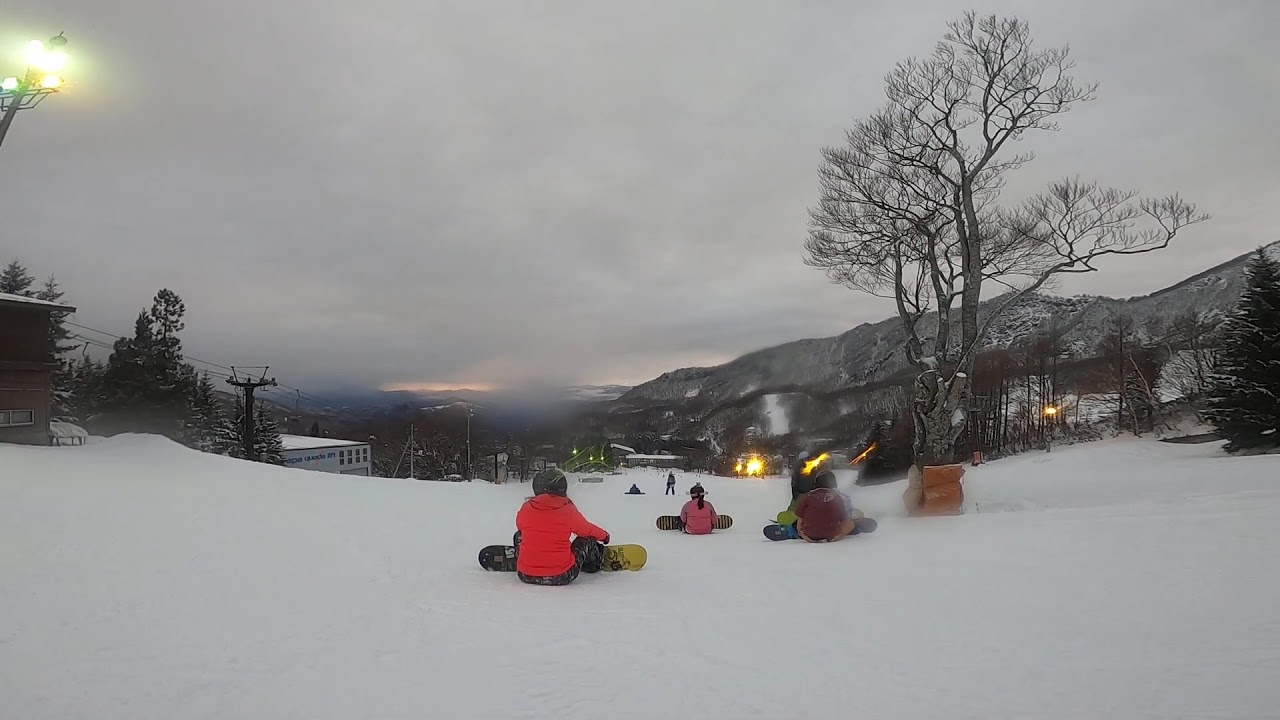In this color photograph taken from a potential GoPro video camera on a snowboarder’s helmet, we see a snowy landscape as the sun prepares to set. The scene captures three young children, approximately 10-12 years old, seated on a snow-covered slope. They sit with their legs crossed, their snowboards laid out in front of them, possibly taking a break from their snowboarding activities. Each child is wearing a helmet and distinctively colored jackets: the child on the left sports a bright orange jacket, the one in the middle is in pink, and the one on the right is in red. Next to the child in the red jacket is a tall, leafless tree with some white and orange material wrapped around its base. The overcast sky adds to the cold and wintry atmosphere, and the horizon reveals the silhouette of distant mountain ranges. Additionally, glimpses of buildings peek from the left side of the image, reinforcing the setting as a dedicated area for snowboarding or skiing. The overall mood is serene yet lively, capturing a moment of rest amidst a day of winter sports.